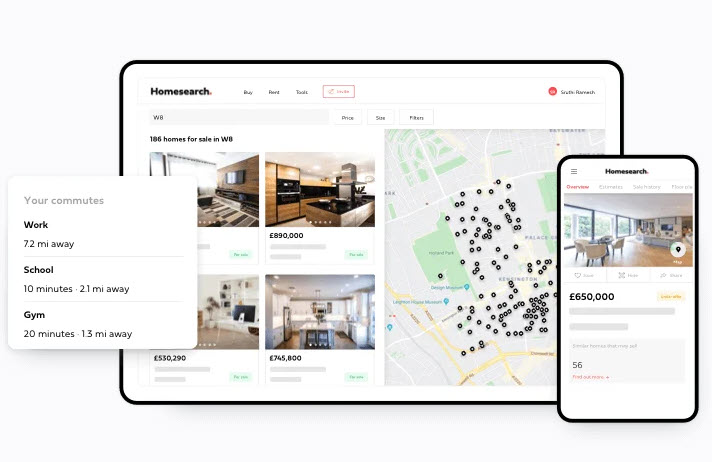In this image, we see a detailed screenshot presented against a white background. On the left, there is a small white box providing information about various commutes. It states, "Your Commutes: Work - 7.2 miles away, School - 10 minutes, 2.1 miles away, Gym - 20 minutes, 1.3 miles away." This box is positioned in front of a larger screenshot that occupies the upper left corner of the image.

In the larger screenshot, we notice a home search interface indicating that there are 186 homes for sale. To the right of this interface, there is a detailed map. The map features a gray background with various sections marked in green to represent parks. Roads are highlighted in yellow, gray, and white, with black circles denoting the locations of available homes.

Within the map, Highland Park is discernible as one of the green areas, with Kensington situated to the right (or east) of it. Kensington appears to be the primary area where most of the homes for sale are concentrated. The overall composition of the image is informative, providing a clear visual representation of the commutes, available properties, and geographic layout of the neighborhoods in question.